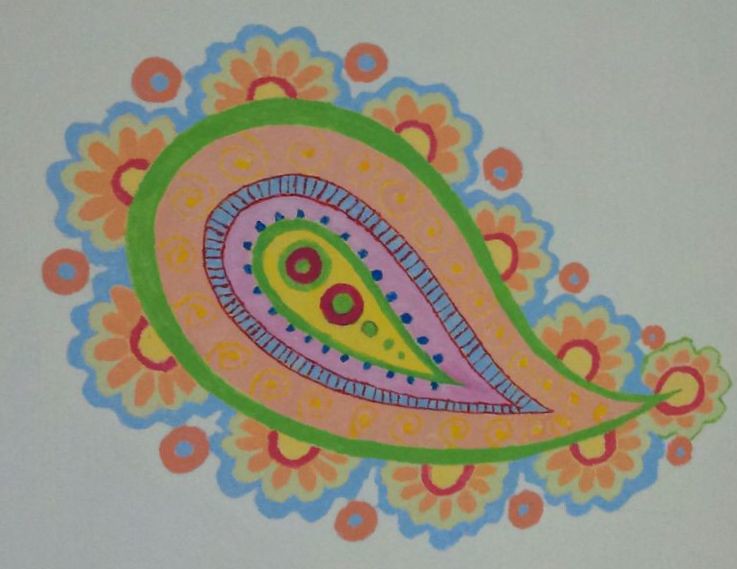The image is a meticulously crafted, colorful drawing on a white sheet of paper, created with markers. The overall form is a teardrop shape, slightly wider than it is tall, oriented with its pointed end directed toward the lower right-hand corner and the broader end facing the upper left-hand corner. This intricate design features a multi-layered pattern resembling raindrops within raindrops, akin to a nesting doll configuration.

Starting from the center, the teardrop is filled with various colored sections and detailed patterns. At the core, a yellow teardrop holds three intricately outlined green dots. Surrounding this is an alternating sequence: an orange layer, then a blue segment with red outlines, followed by pink with blue dots, another green outline, and finally yellow, which includes green concentric circles with red dots.

Enveloping this structure is a medium green outline, around which is a layer of blue dots evenly dispersed. This is further encased by a light green border followed by a pink outline with red detailing. Expanding outwards, a peach-colored section features subtle yellow swirls, encircled once more by a light green line.

The exterior edge of the teardrop is adorned with flowers that have a yellow center, red rim, and peach-colored petals outlined in green and blue. Between these flowers, blue dots with peach outlines elegantly fill the gaps. The entire background of the image is a medium gray, making the vibrant colors of the design prominently stand out.